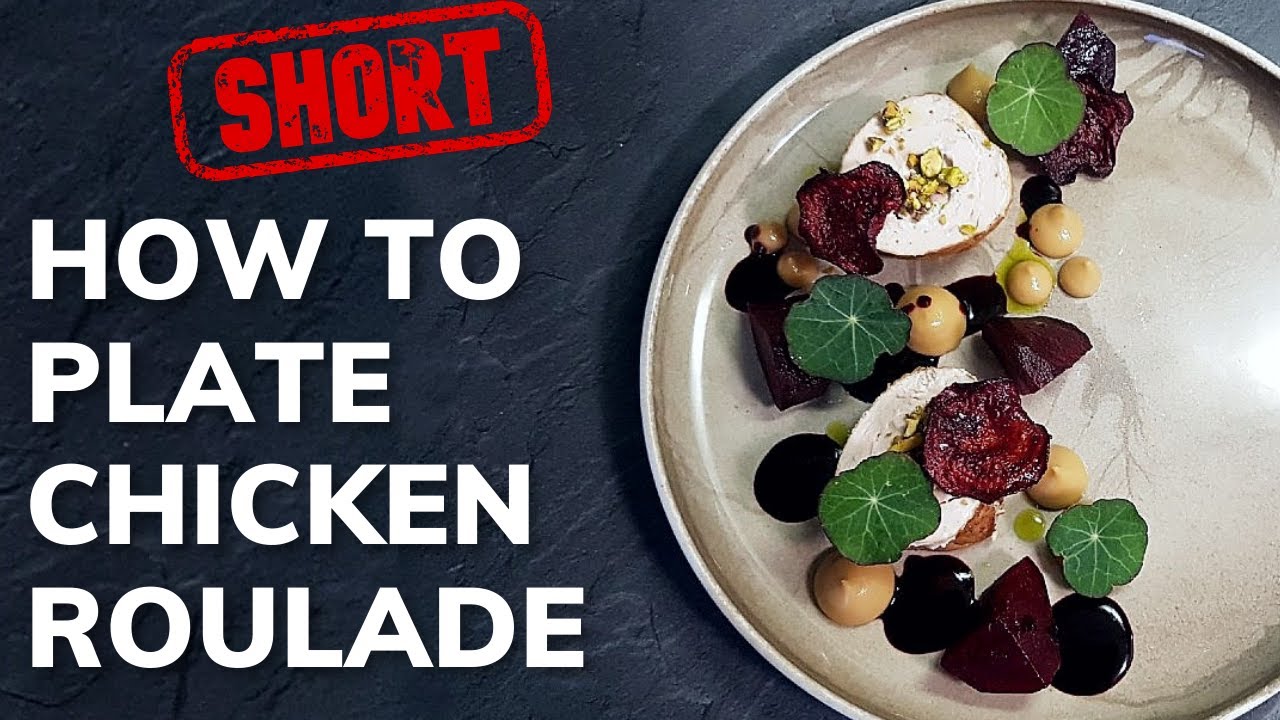This photograph, possibly the start of a video tutorial or blog post, features a meticulously designed guide on "HOW TO PLATE CHICKEN ROULADE." The main text is displayed prominently in large white capital letters, with "SHORT" positioned in the top left in bold red block letters outlined in red. The backdrop is a dark grey marbled texture, adding a sophisticated touch. To the right, a light brown, almost grey earthenware clay plate with curled edges showcases a beautifully plated chicken roulade. The dish includes sliced chicken roulade adorned with what appears to be dried red beet slices, a couple of piped tan-colored sauce dollops, and decorative green leaves. Additionally, there are elements that might be figs, pistachios, mushrooms, or chickpeas, all lightly drizzled with olive oil, presenting a visually appealing gourmet meal.